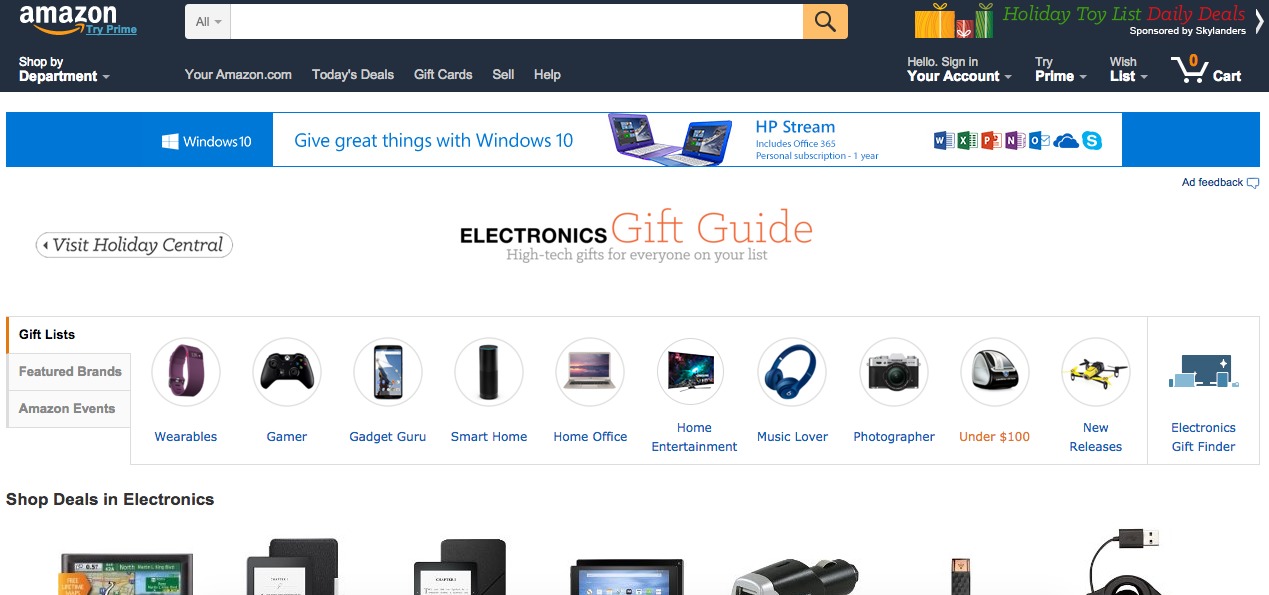The image is a detailed screenshot from the Amazon website, displayed against a white background. In the upper left corner, set against a black banner, it reads "Amazon Try Prime, Shop by Department." Next to this, on the right, is the familiar Amazon search bar. Directly beneath these elements, running left to right, are several navigational options: "For Amazon.com," "Today's Deals," "Gift Cards," "Sell," "Help," "Hello, Sign In Your Account," "Try Prime," "Wish List," and a shopping cart icon displaying a count of zero.

Adorning the page above the navigational bar are three brightly colored illustrated gifts in yellow, red, and green, accompanied by the text "Holiday Toy List Daily Deals," sponsored by Skylanders. Further down, on the lower left side of the page, there's a section promoting deals in electronics. Above this, several categories are listed under "Gift Lists, Featured Brands, Amazon Events," including "Wearables," "Gamer," "Gadget Guru," "Smart Home," "Home Office," "Home Entertainment," "Music Lover," and "Photographer." The entire interface showcases Amazon’s efforts to help users easily navigate and find holiday gifts across various categories.